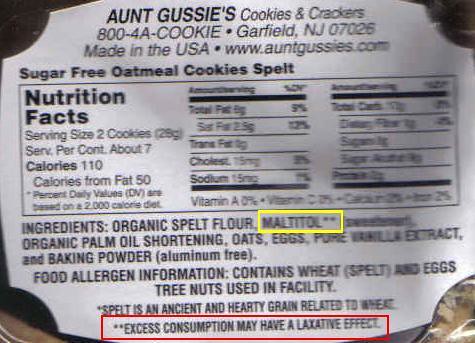The image displays a black and white nutrition label for Aunt Gussie's Cookies and Crackers, a company based in Garfield, New Jersey (07026), with the contact number 800-4-A-COOKIE and their website www.auntgussies.com. The product detailed is sugar-free oatmeal cookies made from spelt flour. The top of the label prominently declares "Made in the USA." Within the nutrition facts section, which is somewhat blurry, it notes that a serving size is two cookies (approximately 26 grams), with about 110 calories per serving, 50 of which are from fat. Total fat, trans fat, and carbohydrate details are included but illegible due to the blur.

Under the nutrition facts, the ingredients list includes organic spelt flour, maltitol (highlighted with a yellow box and two asterisks), organic palm oil shortening, oats, eggs, pure vanilla extract, and aluminum-free baking powder. The allergen information specifies the presence of wheat, spelt, and eggs, and mentions that tree nuts are processed in the facility. An important notice at the bottom, outlined in a red rectangle with two asterisks, states that "excess consumption may have a laxative effect." Additional information explains that spelt is an ancient and hearty grain related to wheat.